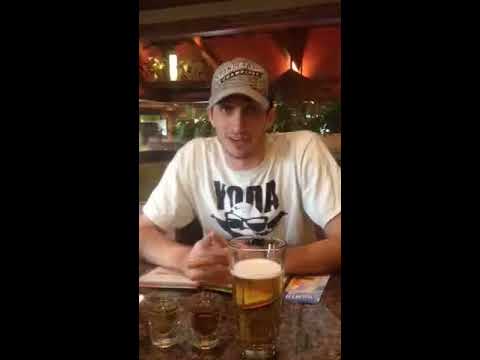A young Caucasian man with short hair, a mustache, and light beard growth is seated at a bar, facing the camera with his fingers clasped together on a mottled brown and grayish-white bar counter. He is wearing a white t-shirt featuring an image of Yoda with sunglasses and the word "Yoda," along with a brown cap. In front of him are three drinks: a large glass of beer and two shots. A book and a pamphlet lie beside the drinks. The bar's background includes greenery, a red wall, and wooden rafters with orange accents. Above his head, there are light sources on the wall and a high shelf, adding to the bar's cozy atmosphere. The man appears to be mid-speech, contributing to the lively scene.